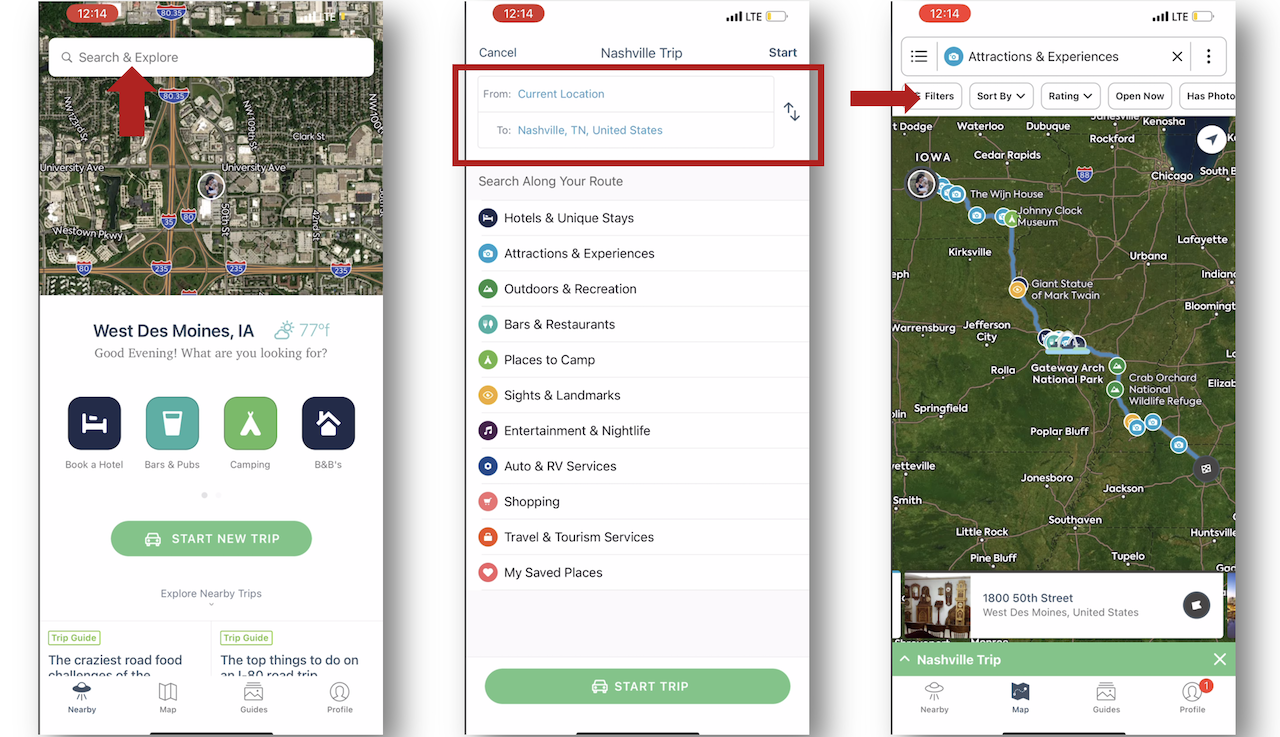The image consists of three distinct snapshots of a navigational driving application. 

**Left Screen:**
- A red arrow highlights the search bar located at the top.
- Below the search bar, there is an option to start a new trip.

**Middle Screen:**
- A red rectangle outlines the top portion of the screen.
- This section displays the 'From' and 'To' locations, presumably as an example. 
- The title "Nashville Trip" is prominently displayed at the top.

**Right Screen:**
- A red arrow directs attention to a button labeled "Filters."
- Central to this screen is a map showcasing a route in light blue.
- Several destinations are marked along this route.
- At the top, a search bar is labeled "Attractions and Experiences."